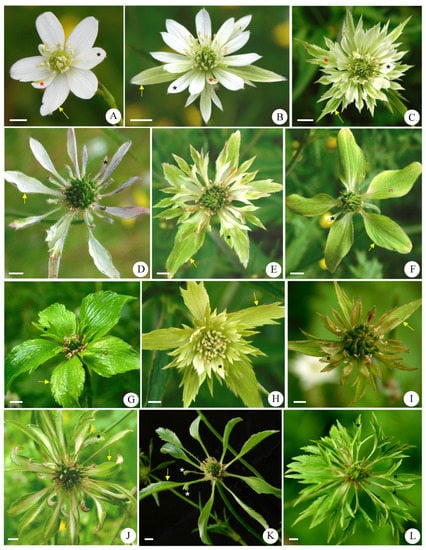The image is a detailed poster with twelve square sections, each containing a distinct flower, labeled from A to L. Each flower has a unique combination of petal shapes and colors, drawn against various backgrounds. Most backgrounds feature green plant life, giving a natural ambiance, except for K, which has a black background. 

- **A**: White petals with greenish-yellow insides.
- **B**: More numerous white petals with green centers.
- **C**: Spiky white petals and a green center.
- **D**: Sparse, skinny white petals with a green interior.
- **E**: Spiky green and white petals with a green inside.
- **F**: Green petals accented with yellow.
- **G**: Green leaves and a brown center.
- **H**: Brownish-green petals.
- **I**: Reddish-green petals with a green interior.
- **J**: Similar to I, with reddish-green petals and a green center.
- **K**: Sparse green petals against a black background.
- **L**: Numerous green petals.

All these flowers are drawn within white-outlined boxes, each unique in its petal structure and coloration, showcasing a variety of botanical designs.